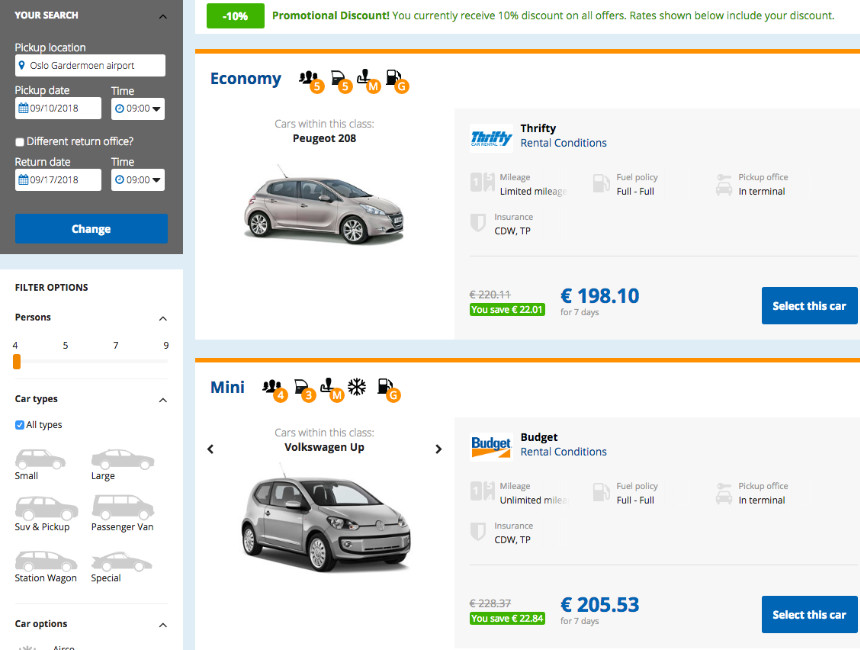This is a detailed caption for the cleaned-up image:

---

The screenshot showcases a promotional offer page from the website "people.com." The background is predominantly white with elements of green and blue.

At the top, there's a green rectangle highlighting a "negative 10% promotional discount," indicating that the user currently receives a 10% discount on all offers. Below this, there's a note that specifies, "Rates shown include your discount."

Within the offer section for rental cars, specific details for an economy class vehicle are provided. This vehicle is a Peugeot 208 (corrected spelling: PEUGEOT). The image includes a four-door minivan icon, emphasizing the type of car.

Key rental conditions are listed as follows:
- The rental term is for seven days.
- The original price of €222.11 is struck through, showing a discounted rate of €198.10.
- This results in savings of €22.01, prominently displayed in a green rectangle.
- Additional details include mileage (with a limited mileage policy), fuel policy (full-to-full), and insurance coverage (CDWTP).
- The pickup location specified is at an office and terminal.

Icons representing the vehicle's features include an "M" and a gas pump, likely indicating manual transmission and fuel-related details. The people icon with "four" signifies that the car can accommodate four passengers.

Lastly, a blue rectangle with white text states, "Select this car," inviting users to choose this particular offer.

---

This caption provides a thorough and detailed description, encapsulating all of the essential elements present in the screenshot.